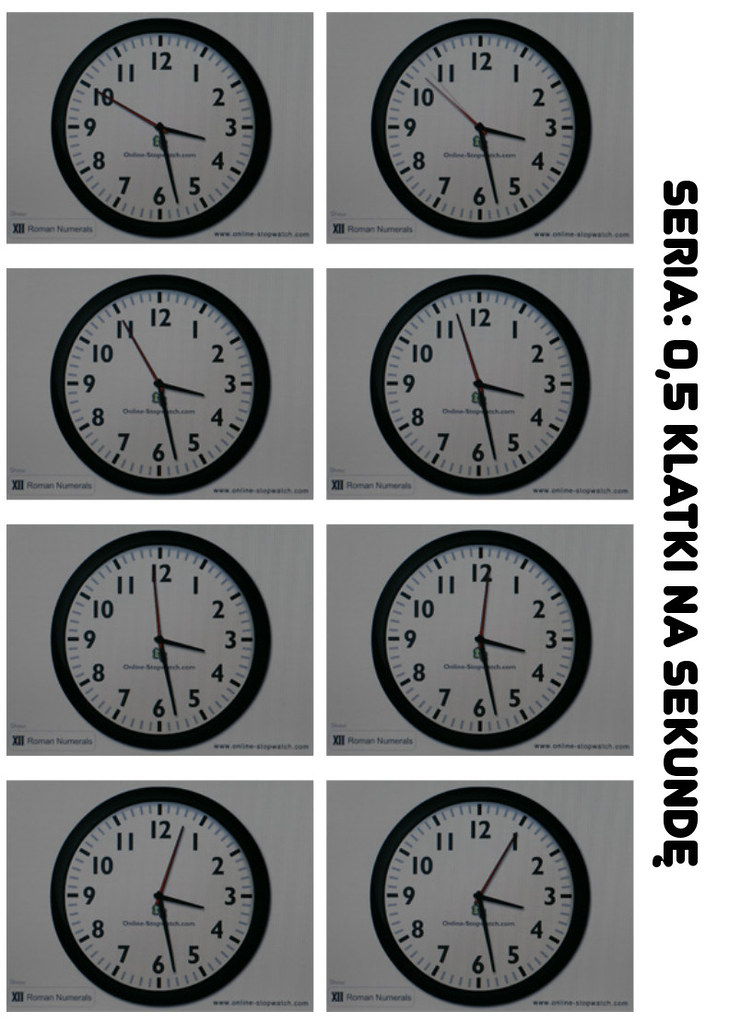This black-and-white image features a set of eight photographs arranged in a 4x2 grid, where each row displays two clocks. The clocks, positioned side-by-side, show slight variations in time, particularly in the placement of the second hand. 

On the far right side of the image, inscriptions in black text run vertically, requiring the viewer to tilt their head to read them. The text reads: "Siri: 0.5, clacky, na, secunda." 

Zooming in on the clocks, it is noticeable that the hour hand on the top row of clocks is near the 3:25 to 3:30 mark. The second hand changes position slightly on each successive clock from top to bottom. 

For instance:
- The first clock’s second hand is close to the 10-second mark.
- The second clock’s second hand points between the 10 and 5-second marks.
- By the time we reach the third clock, the second hand is slightly past the 5-second mark.
- Finally, on the bottom-most clock, the second hand appears to be around the 1 or 5-second mark, indicating a gradual progression in time across the sequence of clocks.

This detailed arrangement and subtle progression suggest a careful study of time intervals and differences in the depicted clocks.